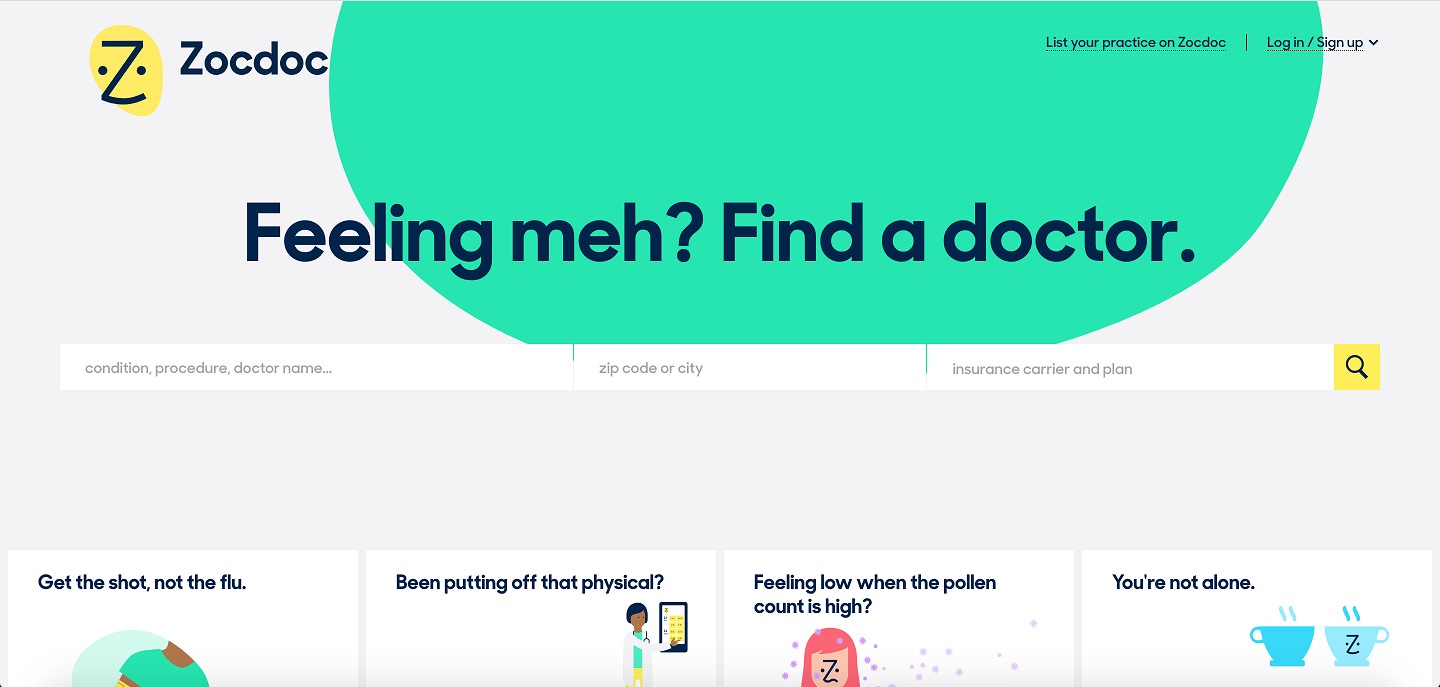**Detailed Caption for ZocDoc Webpage Screenshot:**

The screenshot captures the homepage of the ZocDoc website. In the upper left-hand corner, the ZocDoc logo is prominently displayed, highlighted in yellow, and accompanied by the ZocDoc name. In the upper right corner, there are options to "List Your Practice on ZocDoc" and a "Login/Sign Up" button. The background features a pleasant green blob design at the top, adding a touch of color.

The center of the page is dominated by a bold and inviting message: "Feeling meh? Find a doctor." This call to action is followed by three essential text boxes for users to fill in, making the search for medical professionals simple and intuitive. The first text box prompts users to enter a condition, procedure, or doctor's name. The second box is for entering a zip code or city, and the third box requests the insurance carrier and plan information. To the right of these text boxes, there's a magnifying glass icon indicating the search function.

At the very bottom of the page, partially visible, are four informational boxes with text and icons. The first box, titled "Get the shot, not the flu," encourages vaccination. The second box, with the text "Been putting off that physical?" is a reminder for users to schedule their routine check-ups. The third box asks, "Feeling low when the pollen count is high?" targeting individuals affected by allergies. The fourth box reassures users with the message, "You're not alone," likely addressing mental health or community support resources. Each of these boxes includes unique icons to visually represent the message.